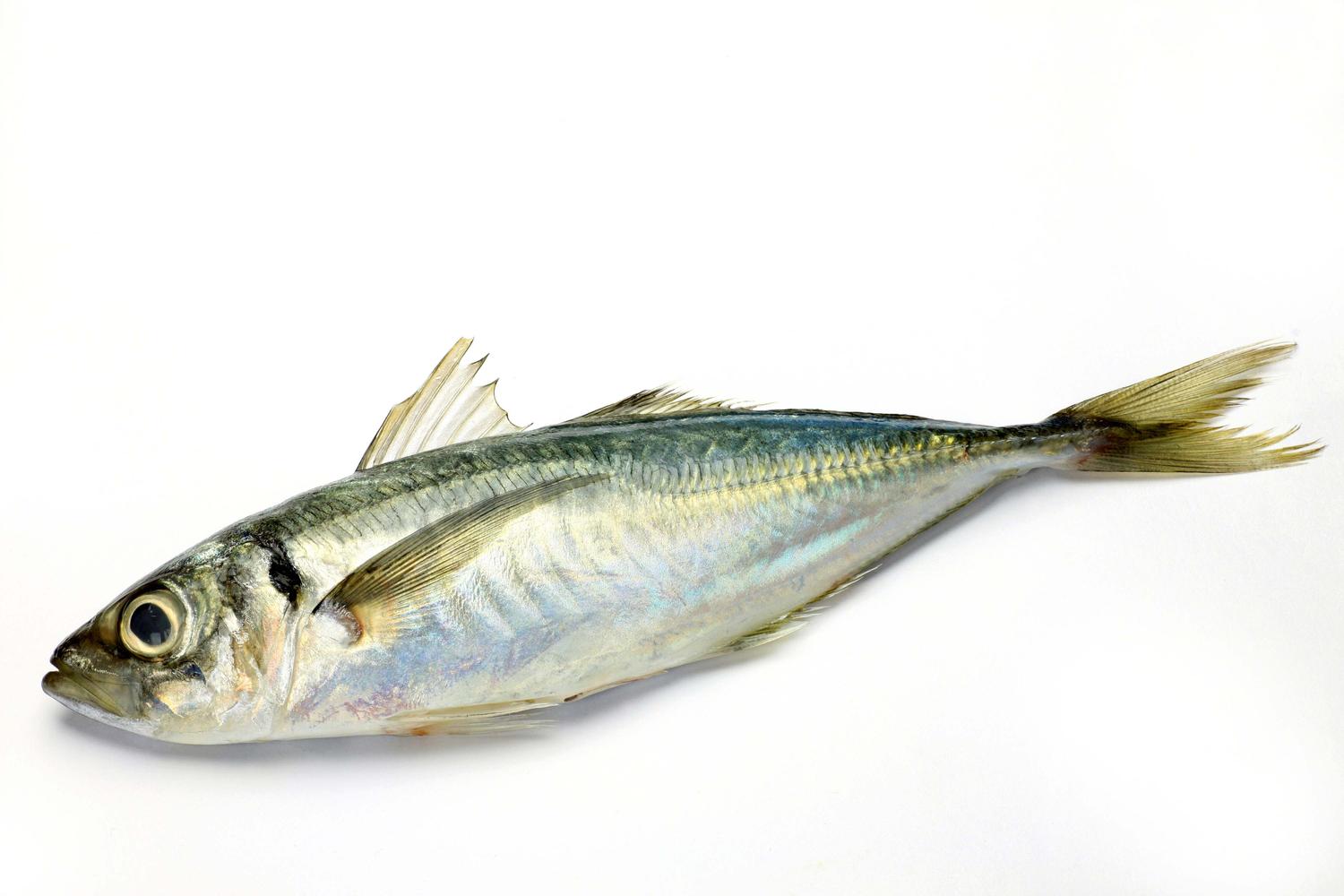The image is a detailed close-up photograph of a single fish, specifically a tuna. The fish is laid out on its side on a solid white surface, with its head pointing towards the lower left corner of the image and its tail sweeping back to the center-right. The background is entirely white, providing a clear and unobstructed view of the fish. The fish has a silvery body with a slight bluish tint and transparent fins. Its black, round eye and open mouth are clearly visible. The overall image is brightly lit, likely by natural lighting or an overhead light source from the camera, making the scene very clear. The photograph captures the fish out of water, emphasizing its shiny scales and sleek form. There are no other objects, text, or watermarks in the image, focusing all attention on the fish itself.